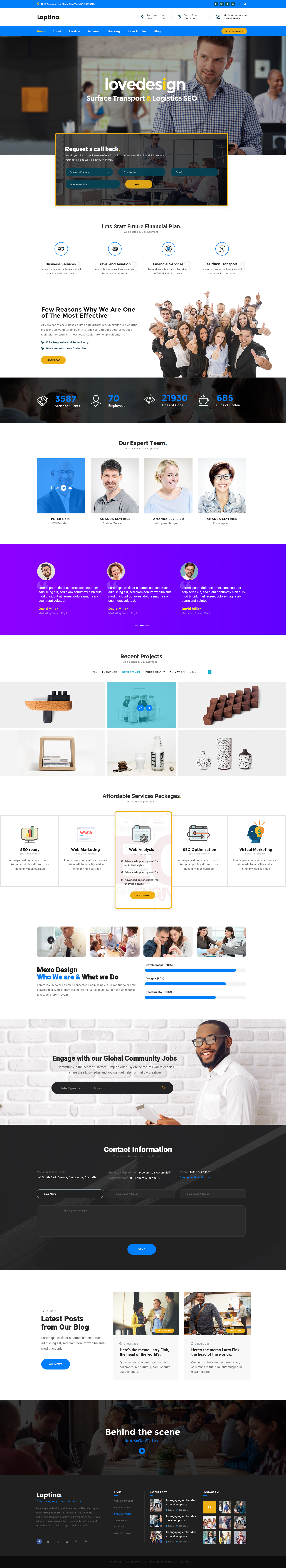This image is a collage featuring several groups and individual portraits against a dynamic backdrop. The overall composition is blurry, and the text appears stretched and difficult to read. At the top, prominently written in white text, is the phrase "Love Design" accompanied by a yellow icon, set against the backdrop of a person wearing a white and blue t-shirt. Below this, the center of the image showcases a group of people, followed by individual portraits beneath. At the very bottom, the image footer has a solid black background with the text "Bring the Love" also in white font. The visual elements and text come together to create a vibrant and intricate design, despite the clarity issues.